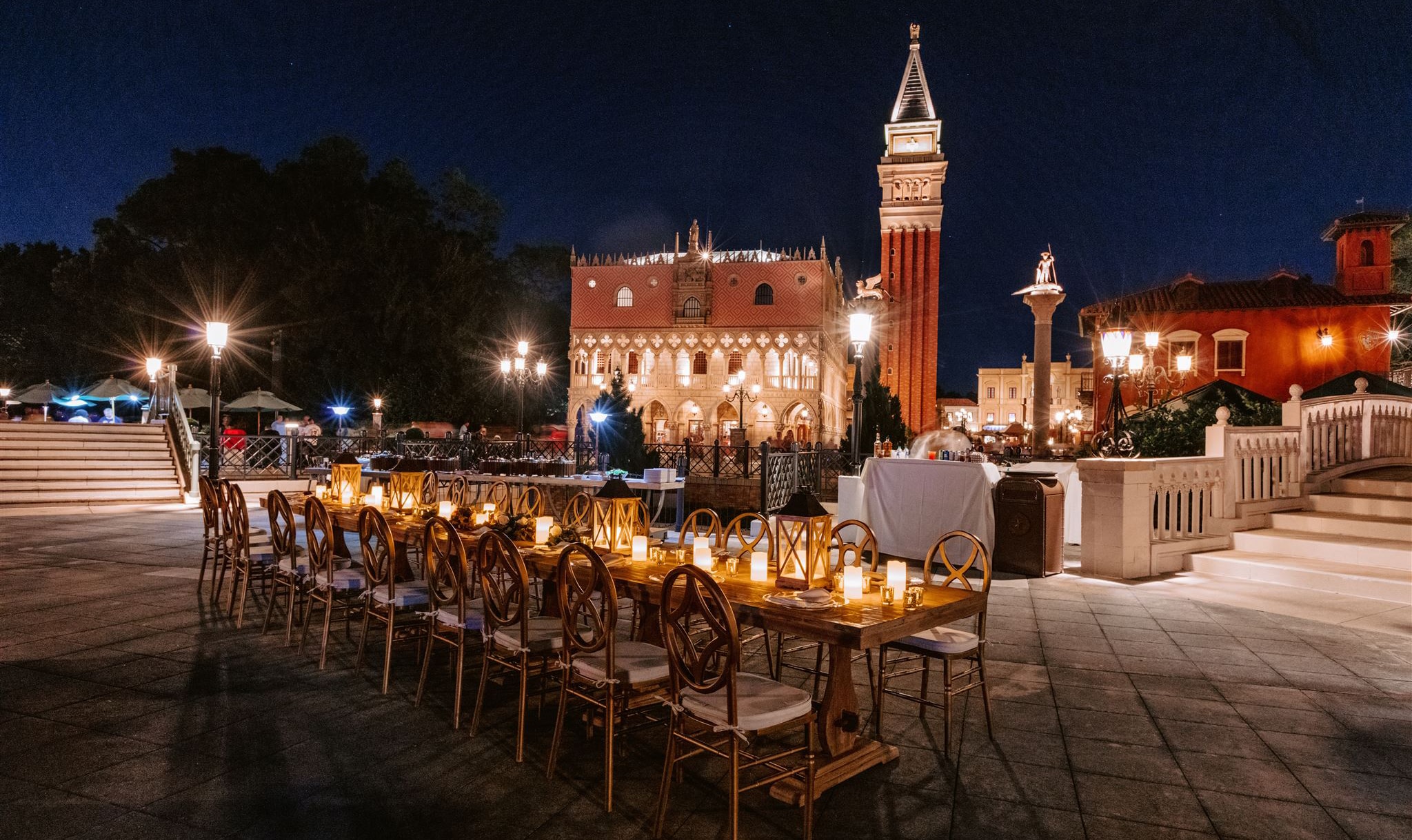The image captures a lavish outdoor dinner setup at night, with a prominent long wooden table and roughly 20 matching wooden chairs arranged along its sides. The table is adorned with candles and illuminated lamps placed along its center. The setting is well-lit despite the dark blue sky, creating a striking contrast against the beautifully illuminated buildings in the background, including what appears to be a grand cathedral. Streetlights and lampposts contribute to the ambient lighting, enhancing the warm, inviting atmosphere. The scene includes a large staircase towards the back left, leading to a bridge that connects to another elegantly lit building. A few trees are scattered in the background, and some people are seen walking and gathering around tables under canopy tents. The entire arrangement suggests a fancy dinner party, perfectly staged but not yet occupied by guests.